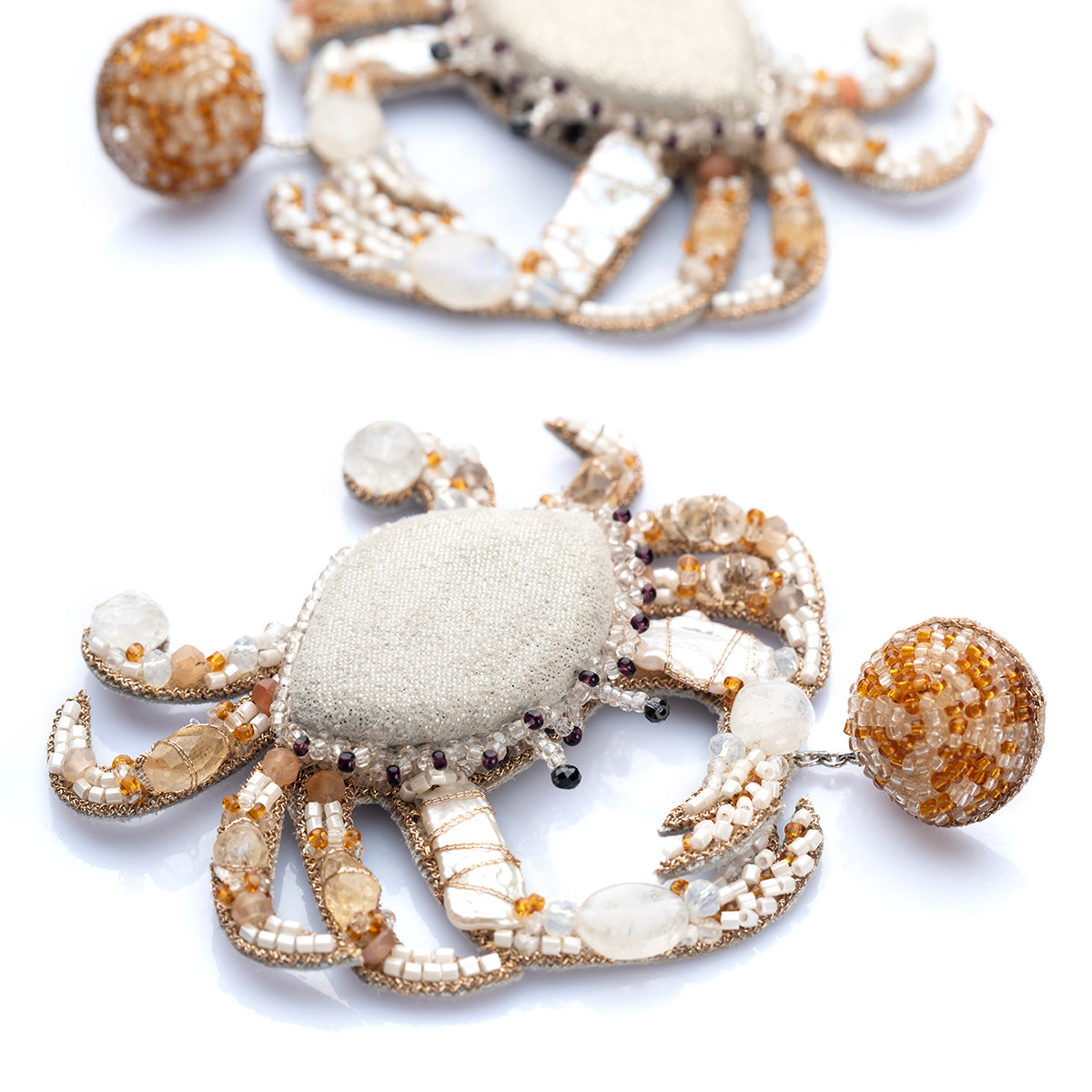The image features two intricately designed crab-shaped jewelry pieces, likely brooches or pins, viewed from above. The crabs are adorned with various gemstones and beads, each showcasing exquisite craftsmanship. The crab at the bottom is more clear and detailed, while the one at the top center is slightly blurry but appears identical or very similar in design.

The lower crab's body is mainly white, bordered by clear and black rhinestones. Its eight legs are adorned with an array of gemstones in shades of white, tan, orange, yellow, and cream, varying in size and adding a texture of opulence. The claws, which are visibly attached, feature smaller gemstones and intricate detailing. One front claw is connected to a metal chain holding a circular item, which is encrusted with tiny gemstones in hues of orange and cream. Additionally, the crab has white antler-like extensions with black beads representing the eyes, adding a lifelike touch to the piece.

The upper crab mirrors the lower one's intricate design but remains less detailed due to its blurry appearance in the image. Both crabs exude a sense of luxury and artistic flair, making the jewelry pieces striking and unique collectibles.